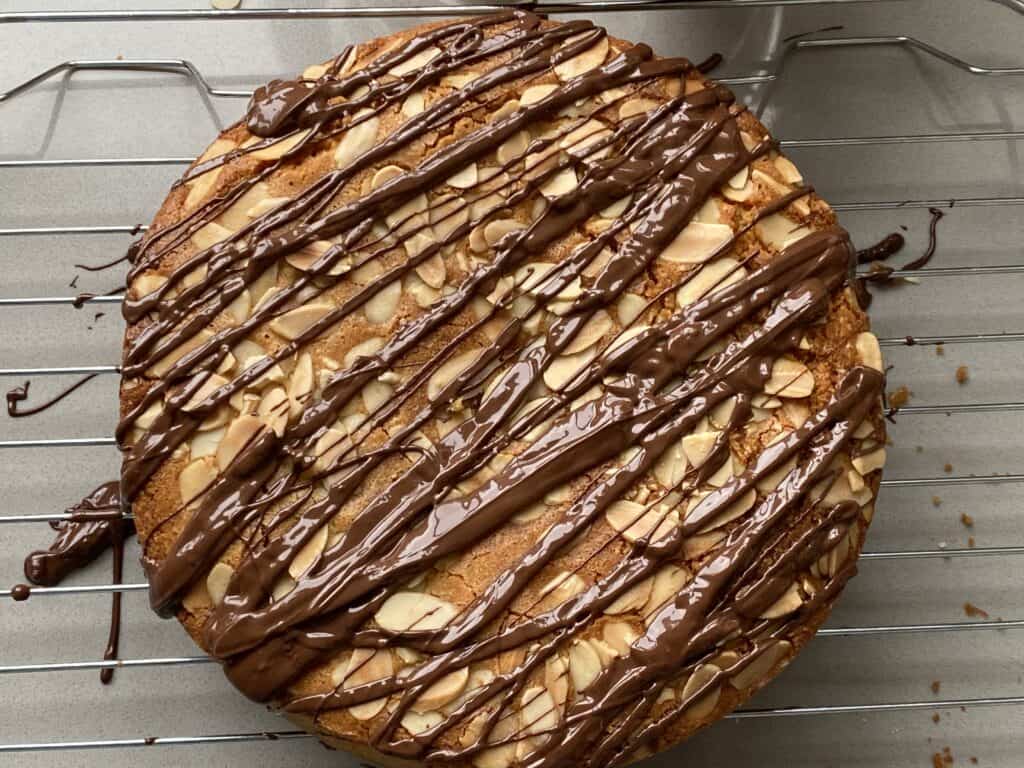The image showcases a tantalizing dessert, viewed from above, prominently placed on a silver cooling rack. The dessert, which might be a large, golden-brown pie or cake, is generously topped with an assortment of nuts, likely walnuts or almonds. Visible streaks of rich milk chocolate are artfully drizzled across its surface, adding to its decadent appearance. Beneath the rack, chocolate has spilled onto another tray lined with parchment paper, enhancing the presentation’s rustic charm. The composition is meticulously captured, emphasizing the dessert's inviting texture and color contrast between the silver and gray of the rack, the warm brown of the baked treat, the light tan of the nuts, and the dark brown of the chocolate. Overall, the image likely depicts the mouthwatering result of a recipe featured on a cooking website.